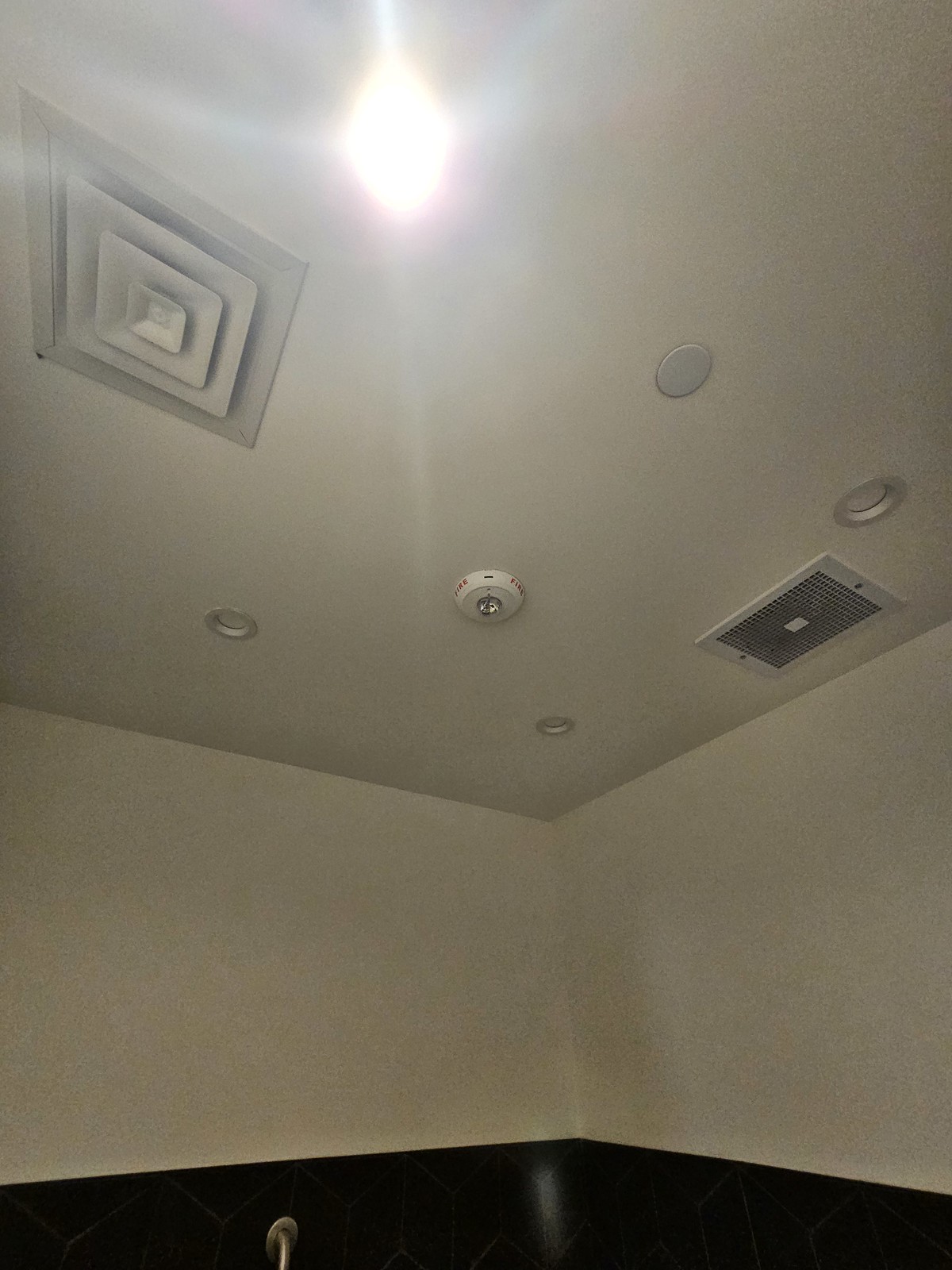The color photograph captures a pristine white room showcasing its minimalist design. Dominated by white walls and a white ceiling, the image reveals the corner where the walls meet, casting subtle shadows that add depth to the scene. Bright illumination emanates from a central light fixture, which appears as an oval shape with radiant streaks, suggesting an overhead light source or a potentially powerful flashlight being shone upwards.

Near the center-left of the image, there is a distinctive white metal exhaust fan with a series of concentric square patterns, adding an architectural element to the otherwise plain ceiling. Another notable feature includes a heater/light combo fixture, often found in hotel settings, suggesting a practical, multi-purpose use of the ceiling space. Supplementing these are recessed ceiling lights, enhancing the room's brightness with a modern touch.

Additional details such as a smoke detector and what appears to be a commercial sprinkler system indicate the room might be part of a hotel or some commercial space, ensuring safety and compliance with building codes. The lower part of the image slightly displays a dark border, which resembles black tile. A partly visible safety grab bar running along the bottom suggests the space could be a bathroom, with functionality prioritized alongside the aesthetic simplicity of an all-white design.